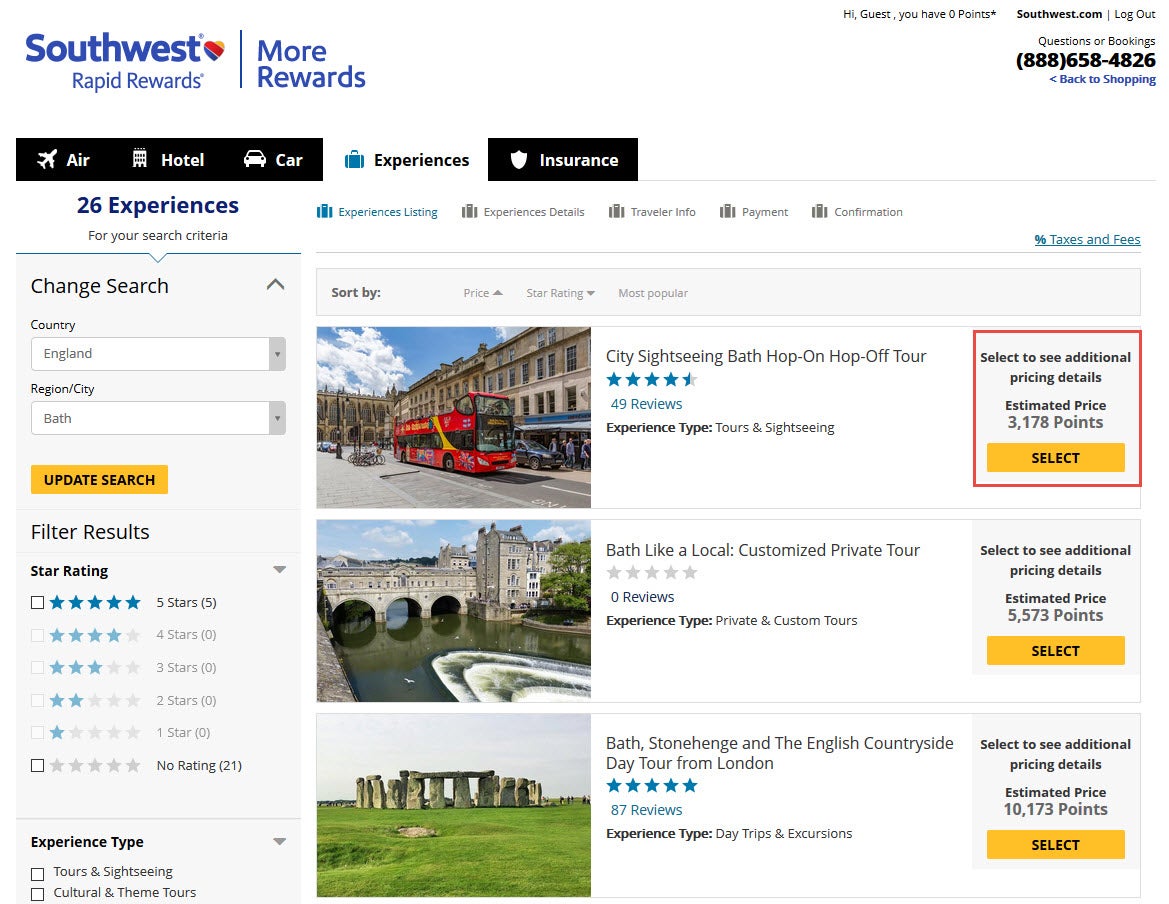This image showcases a webpage from "Southwest Rapid Rewards." Prominently displayed is the Southwest logo featuring a heart in red, white, and blue. The page highlights the message "More Rewards" and offers an 888 contact number for questions or bookings. 

At the top right corner, it reads "Hi, guest, you have 0 points" next to a logout option. A section invites users to "go back to shopping," highlighted in a blue or purple color. Beneath, a black box contains options for "Air, Hotel, and Car," while another black bar provides "Insurance" details. 

The search criteria indicate "26 experiences for your search criteria" with "England" and "Bath" specified. The display includes:
1. **Sightseeing Bath Hop-On, Hop-Off Tour**: An image shows a trolley next to a tall building.
2. **Bath Like a Local: Customized Private Tour**: Features a picture of a historical castle with a moat.
3. **Bath, Stonehenge, and the English Countryside Day Tour from London**: Depicts a lush green landscape with ancient stone ruins.

These curated experiences are aimed at helping travelers explore Bath and its surroundings.